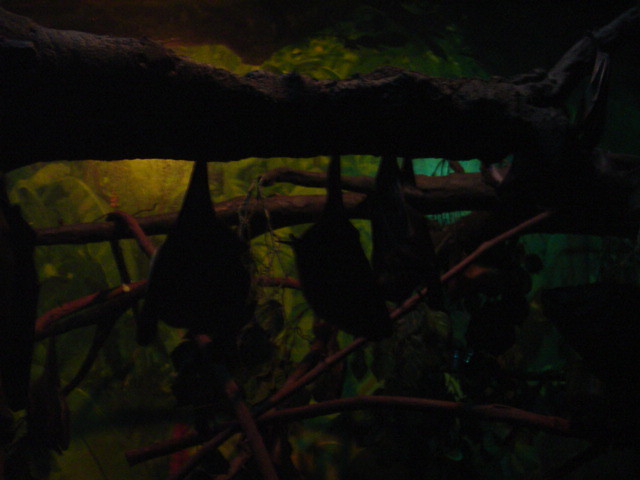The image is very dark, portraying a scene that is quite challenging to discern. At the top of the image, there is a prominent long black log or a thick stick, which has a bumpy texture. Below this main element, there appears to be another thick stick, and further down, yet another stick that seems to branch out. Scattered around these wooden elements, some dark green leaves are visible, adding a touch of natural texture. The background features a light green color, accented by some yellowish lighting effects in the middle area.

Hanging from the main log at the top, there are several shapes resembling bats. These bats have slim black areas tapering into wider bodies, and the barely discernible outlines suggest feet or small paws. They seem to be hanging by their feet from the large branch dominating the upper part of the photograph.

Despite the darkness, there are hints of other objects in the background, which might be additional pieces of wood, possibly some wires or a hose with a reddish hue, though these details are hard to see clearly. The image has a somewhat eerie atmosphere, with unclear surroundings that invite speculation about whether it might be in a basement, shed, or even mistakenly interpreted as elements in a fish tank due to the indistinct forms within the darkened scene.